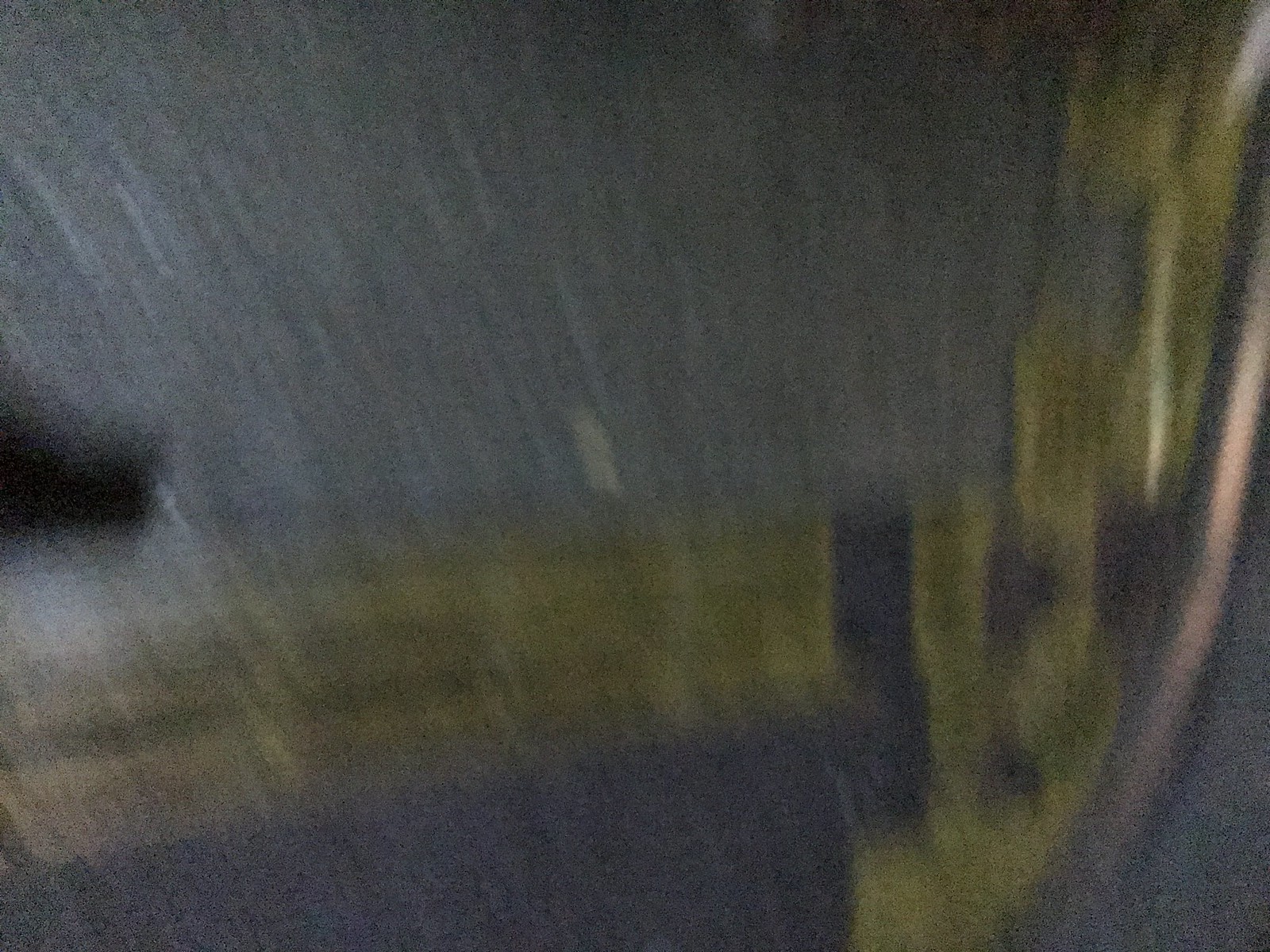A dynamic photograph captures the essence of movement along a gray road. The central focus is a slightly blurred road marked with faint white lines, and a prominent painted line running down the middle, possibly from recent roadwork. On the left side, a blurred section of black transitions into a golden-green hue, spanning a significant portion of the lower center of the image. This vivid color continues in a ribbon-like pattern, interspersed with rectangles of soothing blue that alternate with the golden-green shades. These vibrant colors extend upward along the side of the road. Toward the right-hand side, a streak of lighter pink blends seamlessly into shades of blue, enhancing the sense of speed and motion within the scene. The artistic interplay of colors and the blurred elements suggest movement, perhaps of vehicles or individuals, adding a layer of dynamism to the overall composition.